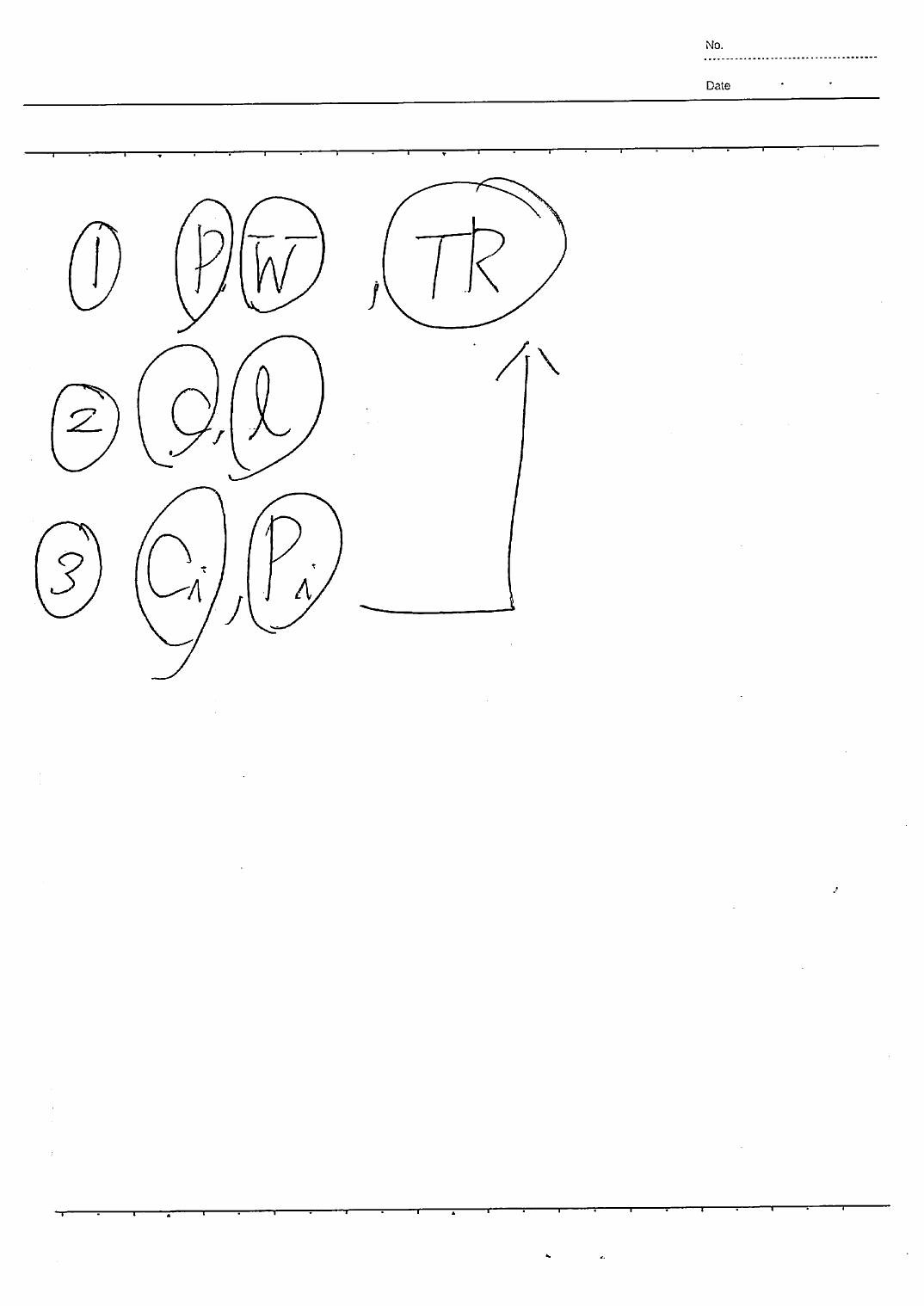This is a large scanned image of a white piece of paper featuring handwritten text, with structured sections for numbering and dates at the top. The paper has two long black lines below the header to demarcate the initial section from the handwritten content beneath. 

1. At the topmost section, there are designated fields for writing a number and a date, separated by black lines.
   
2. The handwritten content begins with:
   - **First line**: The number "1" followed by "P, W, T, R", each character circled ("1", "P", "W", "T", "R" are all individually circled).
   
3. The next line features:
   - **Second line**: The number "2" followed by "C, l", with the number "2", the letter "C", and a lowercase "l" circled individually ("2", "C", "l" are all encircled). Notably, the lowercase "l" is written in cursive.
   
4. On the following line there is:
   - **Third line**: The number "3" followed by "C, I, P, I". Here, the number "3" and the characters "C", a stylized lowercase "I", "P", and another stylized lowercase "I" are circled individually ("3", "C", "I", "P", and "I" are all circled). 

5. An arrow is drawn from the third line (originating from the circled "P, I") at a right angle, then turns upwards to point towards the circled "T, R" on the first line.

The handwritten text is in black ink against the white background of the paper, with various items circled to indicate their importance or connection.

This detailed description highlights the hierarchical structure and organizational format of the handwritten content on the scanned document.